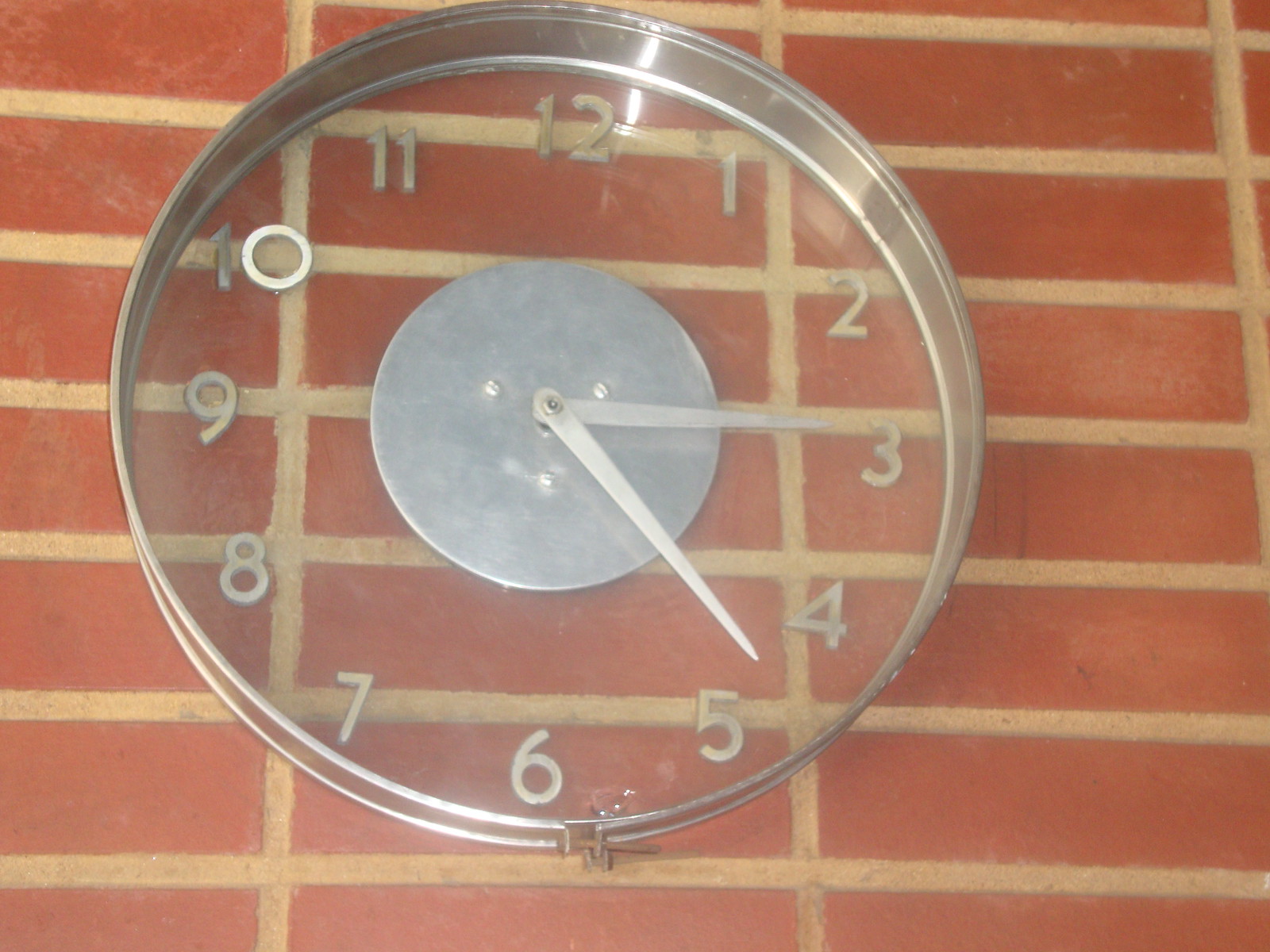A terracotta-colored brick wall with tan grout serves as the backdrop for the image. Affixed to the wall, slightly offset, is an elegant clock. The clock features a sleek silver metal rim, with the front appearing almost wire-like. This rim is complemented by a clear glass cover. The clock face displays standard numerals from 1 to 12, with most numbers in a reflective silver, except for the '10', which appears in a whitish hue. At the center, a silver circle with two small dots marks the location of the mounting screws. The clock’s hands, also silver, indicate the time as 3:23.